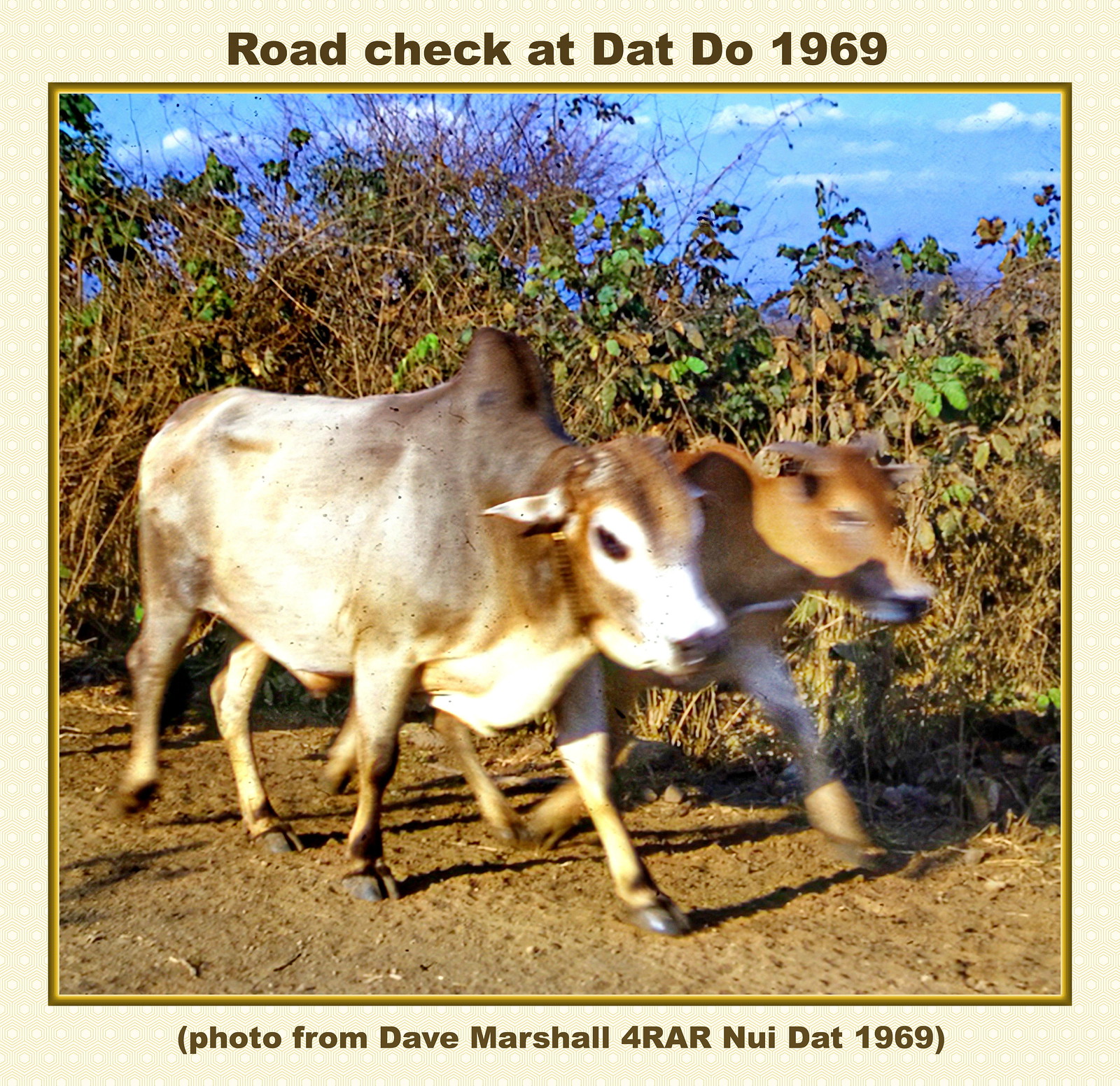The image, titled "Road Check at Dat Due 1969," features two Brahma cows walking side-by-side along a dirt road. The cows, which are primarily tan with some gray and black markings, including around their humps and hooves, are captured against a background of sparse and withered foliage that appears to be suffering from a drought. The landscape shows mostly brown and dead plant life with occasional patches of green. The sky above is lightly cloudy with a serene blue hue. At the bottom border of the image, a caption in parentheses reads, "Photo from Dave Marshall for RAR New Dat 1969."